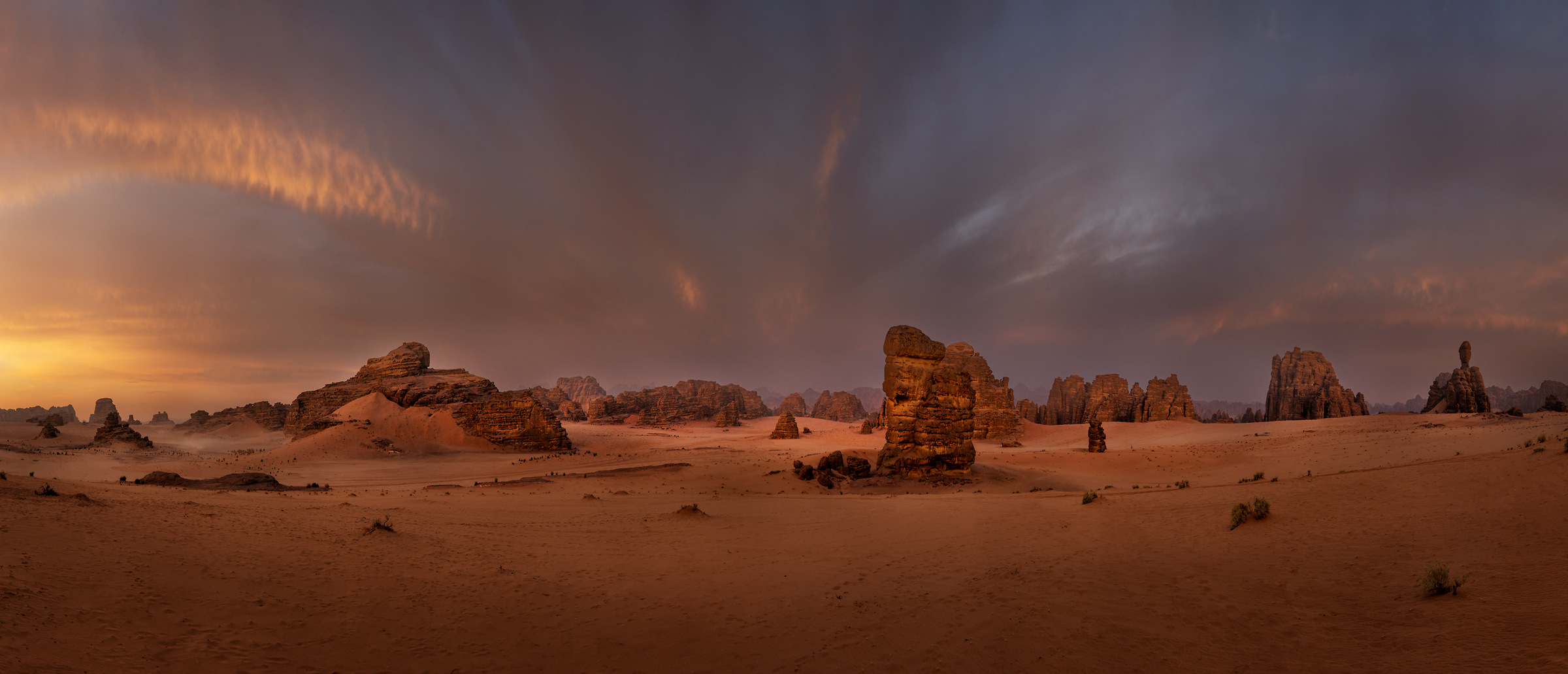This is a detailed, professional photograph of an outdoor desert scene at sunset. The soft, reddish-brown sand stretches across the foreground, interspersed with sparse vegetation and bushes. In the middle of the image, a prominent rocky outcrop resembling a cylinder supports a smaller, darker rock on its top, while to the left, a horizontal rock formation also capped with a single rock adds depth. Scattered across the desert floor, various rocks and smaller formations echo the reddish-brown hue of the sand. The background features an array of rocky structures, with shapes ranging from triangular to rectangular. The sky above displays a dramatic gradient, with a yellow sun situated in the middle left-hand section, casting a soft orange glow on the white clouds. Transitioning to darker hues, the sky evolves from gray to a deep blue, with streaks of clouds reflecting the diminishing light, creating a dusky atmosphere. The overall scene, cast in shadow due to the setting sun, presents a tranquil yet stark landscape ideal for a framed photo.